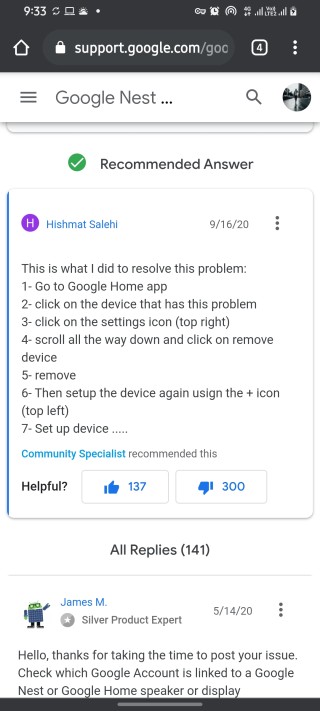Screenshot of a mobile phone screen at 9:33 AM. The phone displays full LTE signal strength and a battery level between 60-80% in the upper right-hand corner. The user is browsing the website support.google.com and has four browser tabs open. The visible tab is a forum thread featuring a recommended answer by Hishmat Salehi on resolving a technical issue. 

The detailed instructions by Hishmat are:
1. Open the Google Home app.
2. Select the problematic device.
3. Tap the settings icon in the top right.
4. Scroll down and click "Remove device."
5. Confirm removal.
6. Re-add the device using the plus icon in the top left.
7. Follow the setup process.

The post notes that "Community specialists recommended this" and poses the question "Helpful?" It has received 137 thumbs up and 300 thumbs down. Below this, the post has garnered 141 replies.